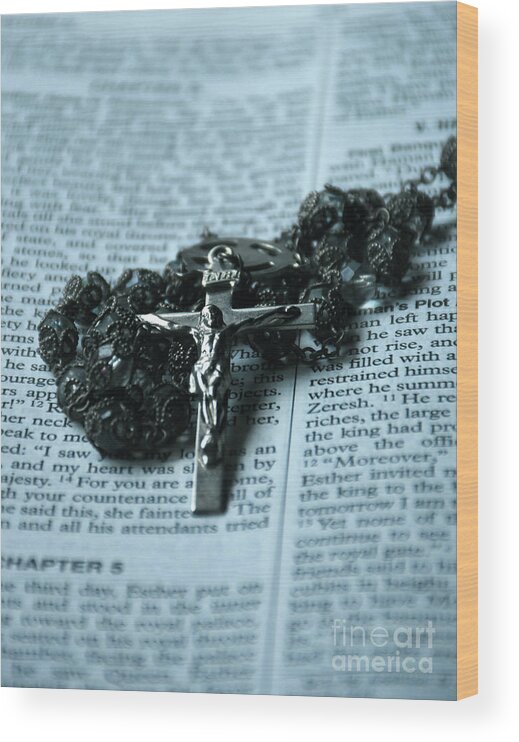This is a detailed close-up color photograph of a silver crucifix with an attached rosary composed of black beads, collectively placed on an open page of the Bible. The rosary beads are jumbled and piled together, making it difficult to make out individual details. The crucifix, positioned in the center of the image, features a detailed depiction of Jesus with his arms outstretched across the cross and legs extending downward. The text on the page is largely out of focus, but a few discernible details include the chapter title "Chapter 5" and the partial word "Zeresh." The overall scene suggests a contemplative and spiritual theme. In the bottom right corner, the text "Fine Art America" is subtly displayed in faded white letters. Additionally, there appears to be a narrow tan stripe along the right edge of the page, contributing to the composition's artistic feel. The main focus of the image is the silver crucifix and the black rosary beads, which stands out sharply against the slightly blurred background.